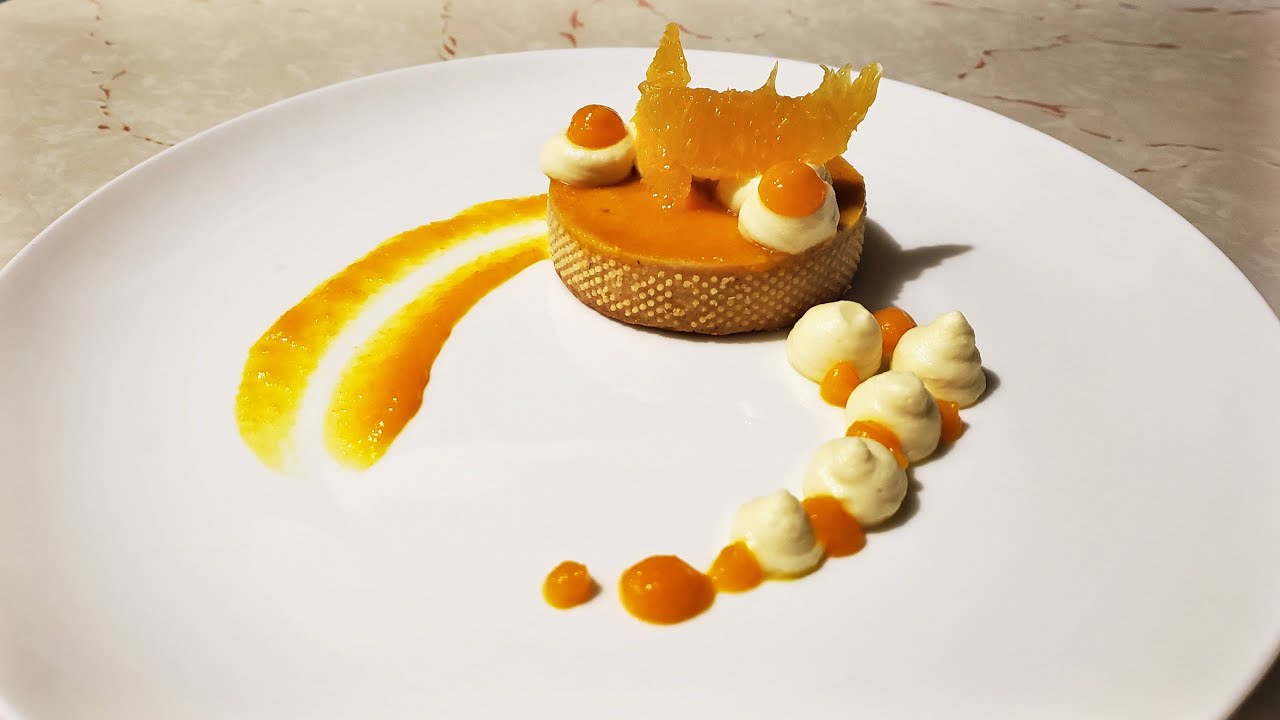This detailed indoor photograph presents a sophisticated, modern dessert on a pristine white circular plate, artistically positioned on a yellow-hued marble surface with intricate striations. The central focus is a petite circular confection, resembling a mini cheesecake or tart, adorned with two segmented orange slices and flanked by two dollops of white cream topped with vibrant orange blobs. To the right, the plate features five more white cream dollops, each paired with an orange dot, while a streak of orange puree artfully stretches to the left. The dessert itself, about an inch thick with an orange surface and white specks, creates a visually striking presentation, indicative of a high-end culinary creation.